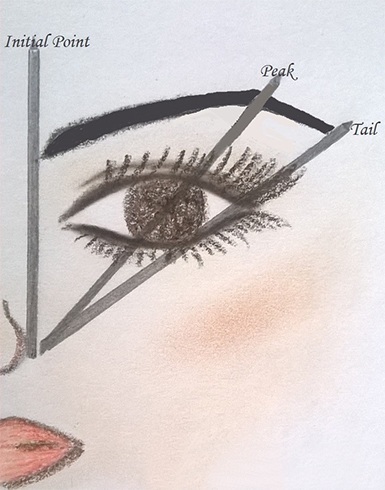The image features a detailed diagram of the left side of a woman's face, primarily focusing on the eye and eyebrow area. The background is light gray, and the image includes a close-up view of her lips, colored with red lipstick, and a partial view of her nose. Overlaid on this partial face is a graph with three distinct lines labeled to guide eyebrow drawing.

A straight vertical line labeled "initial point" marks the beginning of the eyebrow and extends from zero on the y-axis upward, approximately an inch above her eyebrows. Extending from where her eyebrow starts, the middle diagonal line labeled "peak" ends at about a 30-degree angle, aligning with the highest point of the eyebrow's arch. The bottom diagonal line, marked "tail," angles perfectly with her outer eyelashes, indicating where the eyebrow should end.

This instructional diagram also shows the full detail of the eye, including the upper lid, both upper and lower eyelashes, and a brown iris. The visual cues and labels provide a step-by-step guide for accurately drawing an eyebrow, highlighting the initial point, peak, and tail.